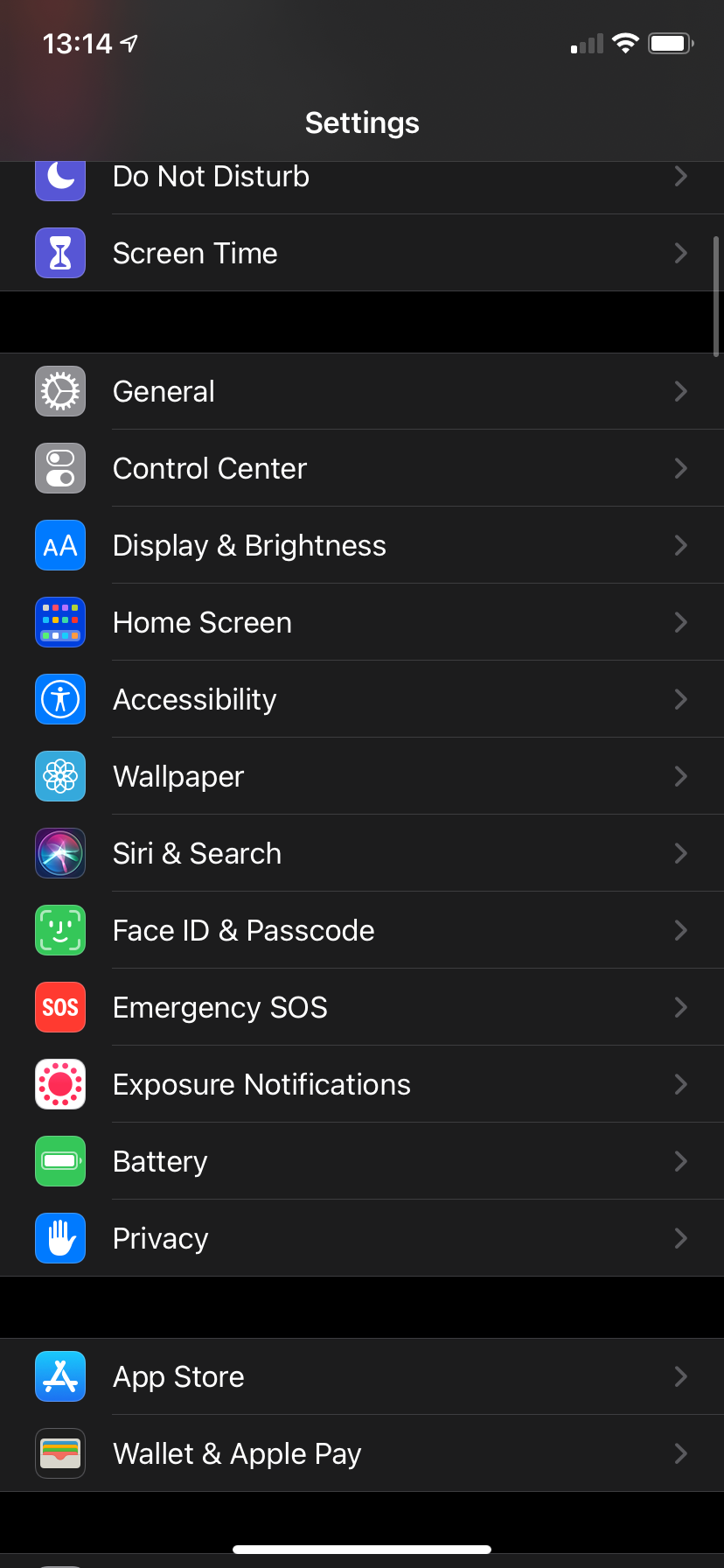A screenshot of a smartphone's settings menu is captured. The top-left corner displays the time as "13:14". In the top-right corner, the phone shows a signal strength of 1 out of 4 bars, a full WiFi signal, and almost a full battery. Below this, the header "Settings" appears.

The settings menu is organized with icons on the left side and their corresponding labels on the right, each entry concluding with a greater-than symbol (">") indicating more options. The listed settings are as follows, from top to bottom:
1. Do Not Disturb
2. Screen Time

There is a black separator area, followed by a gray background for the remaining options. These options include:
3. General
4. Control Center
5. Display & Brightness
6. Home Screen
7. Accessibility
8. Wallpaper
9. Siri & Search
10. Face ID & Passcode
11. Emergency SOS
12. Exposure Notifications
13. Battery
14. Privacy

Another black separator appears, followed by a gray background again with the final options:
15. App Store
16. Wallet & Apple Pay

The layout clearly delineates different sections of the settings, providing a structured overview of the phone's configuration options.